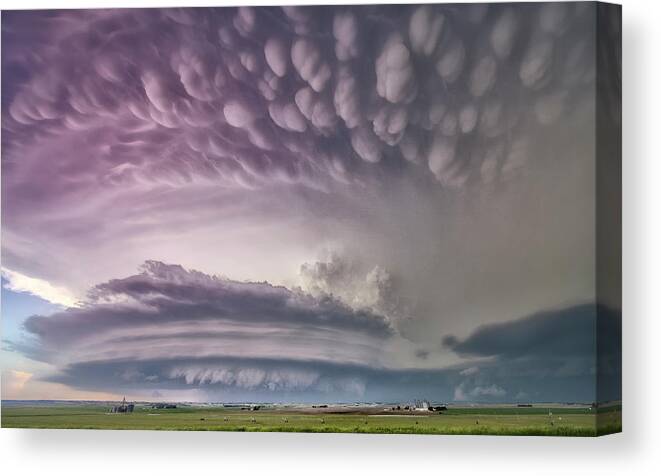The image captures a dramatic and intense landscape, featuring a vast and ominous sky filled with imposing clouds. These clouds, vibrant in shades of light purple, dark gray, blue, and white, resemble segmented cotton balls with a distinct layered formation. Just above the vibrant green grass of what appears to be a sprawling farm field, the clouds manifest in a cylindrical shape, extending downward like tendrils or fingers, suggestive of a potential tornado forming. Beneath this turbulent sky, the ground shows signs of flattened buildings or houses, adding to the chaotic scene. The landscape seems to be taken from a painted canvas, viewed from an angle with a white background, highlighting the dramatic effect of this epic weather phenomenon captured in a still artwork.